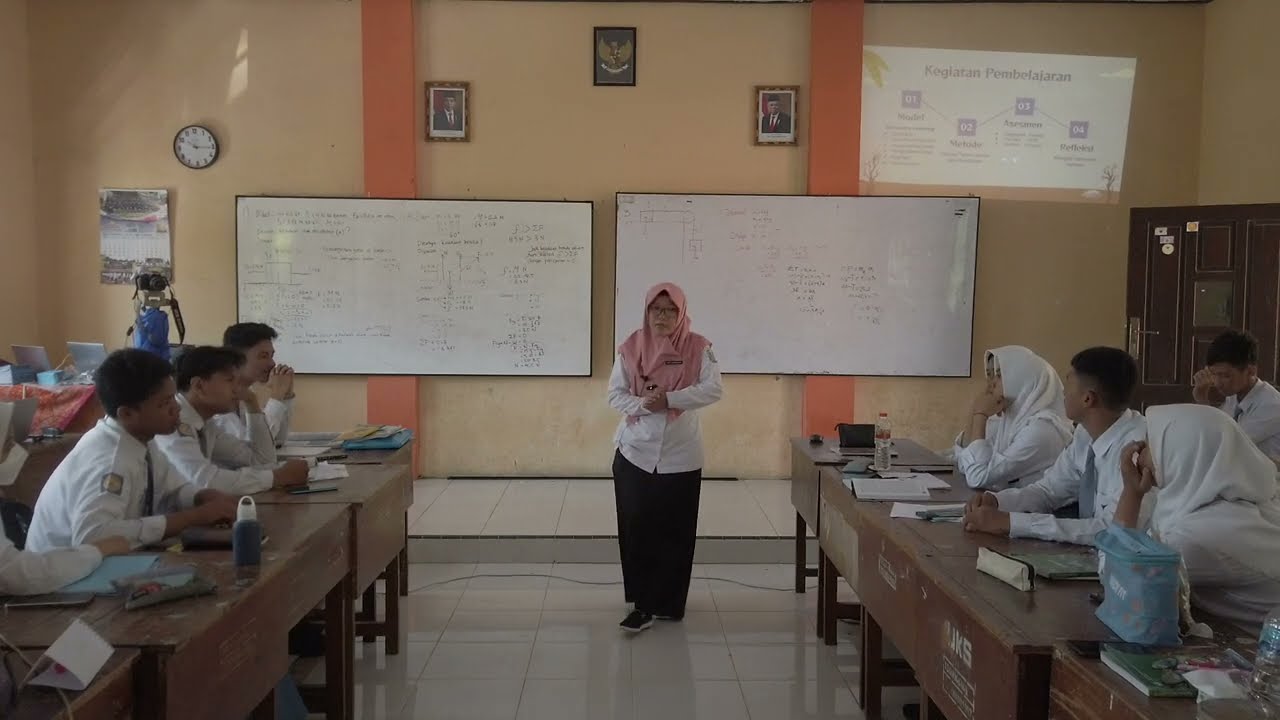The photo shows a classroom setting, likely at the college level as the students appear older. It captures a female instructor, who is likely Muslim and dressed in a white shirt with a headscarf, standing at the center. Behind her are two whiteboards almost filled with mathematical diagrams written in black ink. On her left, there is a row of male students dressed in white uniforms with shirts and ties, suggesting a formal dress code. On her right, there is a diverse row of both male and female students, with the women wearing burkas and also dressed in white. The classroom layout is unconventional, with the instructor in the middle and students seated on either side, suggesting it might be an institution in a Middle Eastern or Asian country, possibly Malaysia.